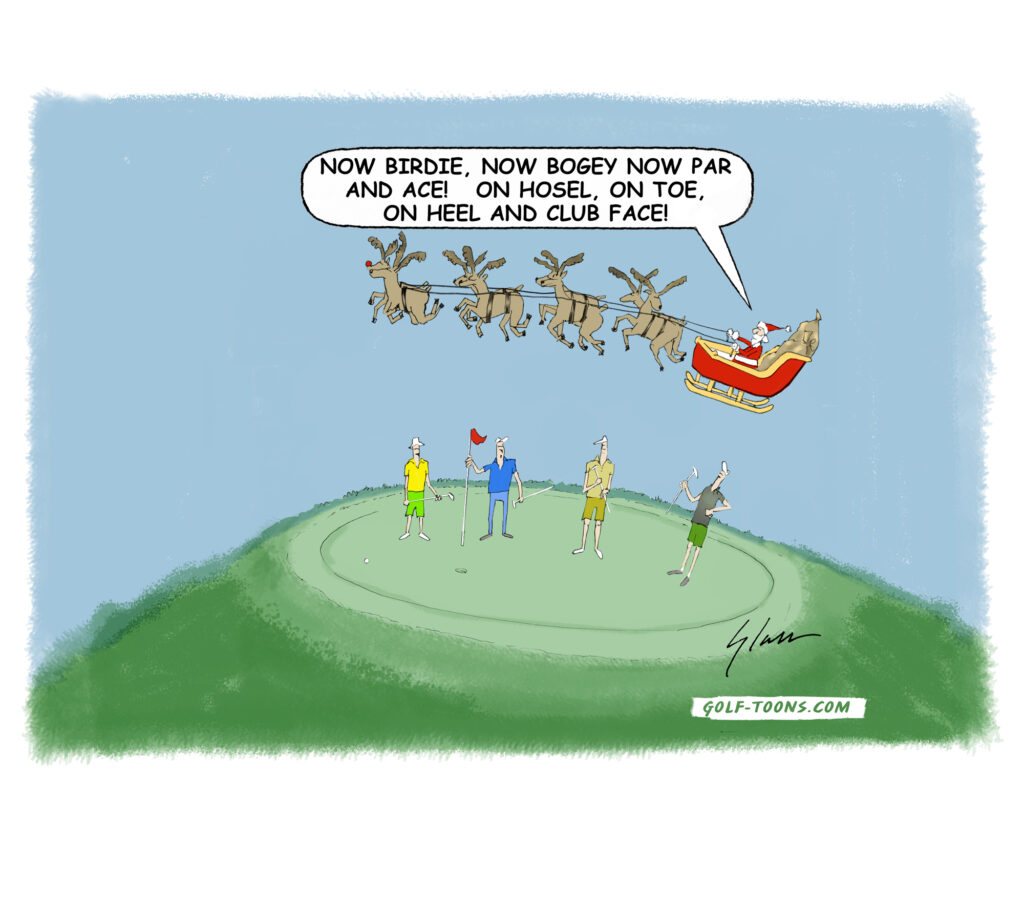In this cartoon image from golf-tunes.com, Santa Claus, dressed in his traditional red suit and pointed hat, is seen flying in the night sky in his sleigh pulled by reindeer. Below him, on a lush golf course with smooth grass on a hilltop and rougher grass on the sides, stand four men gathered around a hole. One golfer holds a red flag attached to a pole. The other golfers are dressed in various outfits, including one in a white hat, yellow shirt, and green shorts, another in blue polo and blue pants, a third in tan shirt with green or orange shorts, and the last in gray and green attire. All of them have their heads tilted upward, looking at Santa as he flies over. In a whimsical twist, Santa is saying, "Now birdie, now bogey, now par, and ace; on hosel, on toe, on heel, and clubface," mixing golf terminology with the names of his reindeer. The cartoon is signed by the artist with an illegible signature, and the domain golf-tunes.com is noted in small white text with gray letters at the bottom right corner.